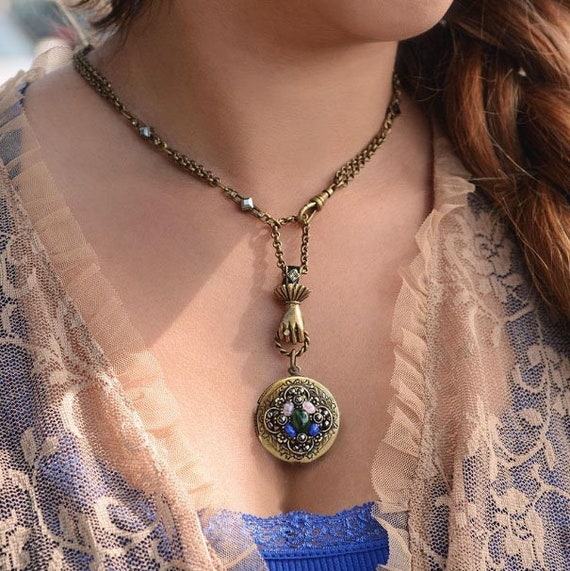This is a detailed, close-up photograph focusing on an ornate bronze necklace worn by a woman. The image captures her chin, neck, and upper chest, with her red auburn hair cascading over her left shoulder. She is dressed in a low-cut blue garment trimmed with lace, revealing some cleavage, and draped in a filmy lace wrap. The necklace comprises a main bronze chain, which connects to a smaller bronze circle chain, followed by a bronze fist holding yet another circle chain that attaches to the pendant. The pendant itself is round with intricate engravings and is adorned with five gemstones—multiple greens, blues, whites, and silver, including a prominent blue gem at the center. This elaborate design highlights the fist clasping the chain, which seems to present the emblem adorned in the jeweled circle, making it the focal point of the image. The setting is well-composed to emphasize the intricate details of the necklace and its unique craftsmanship.